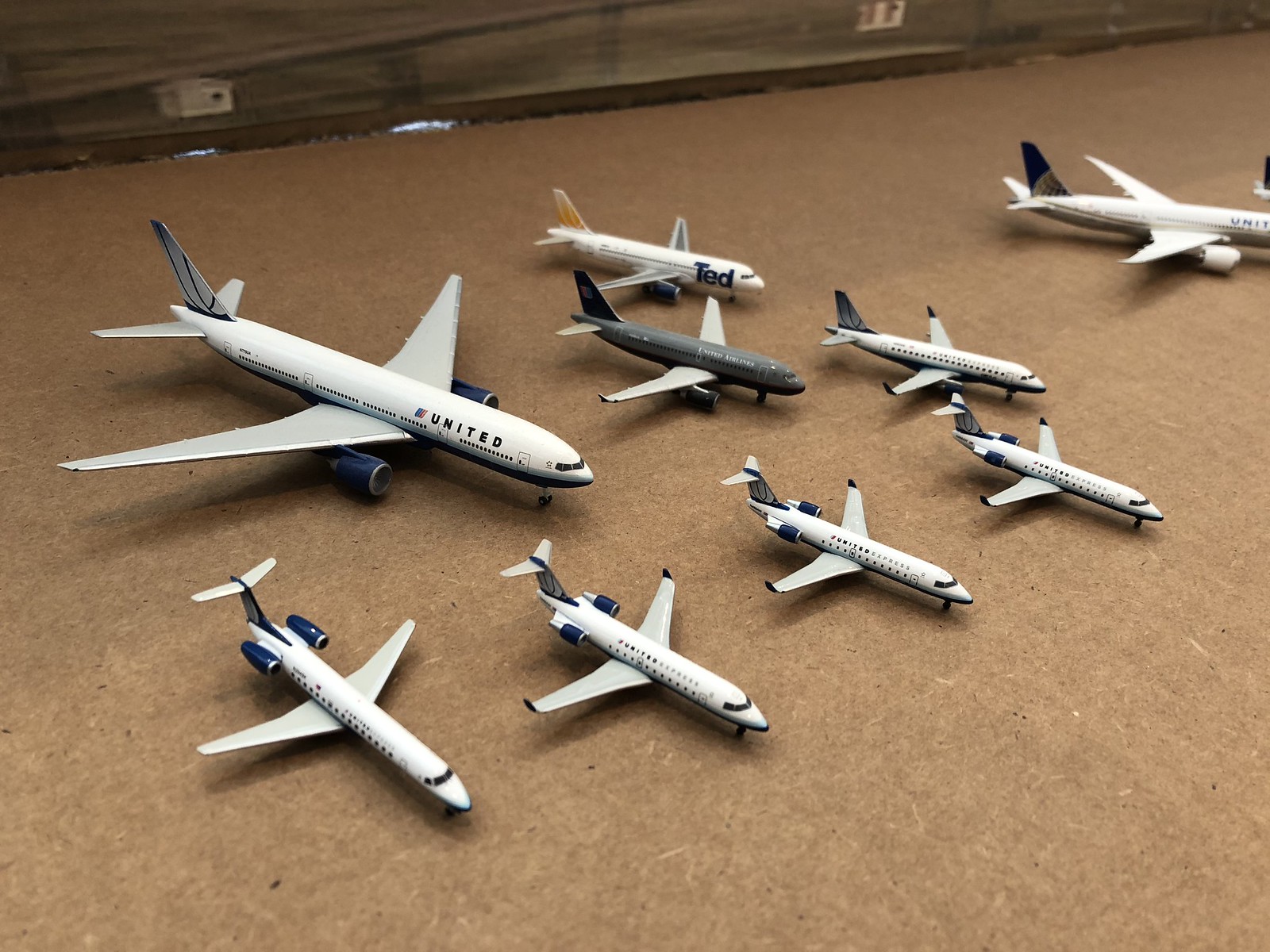In this image, we see an impressive collection of model airplanes displayed on what appears to be a light brown, cardboard-like surface. Dominating the scene is a large, white model airliner bearing the title "United" along with an American flag. This plane has gray wings with blue accents and a tail fin adorned in mostly blue with splashes of white.

Surrounding this prominent model are several smaller planes. Notably, four of these models share a similar design: they have gray wings with blue-tipped stabilizers and tail fins that are largely blue with white highlights. These planes also feature engines near the tail that are partially blue and white.

Another distinct model on the far left shares a similar design to these four but differs with wider back tail fins and completely blue engines. To the right of the large United plane, there is a gray model with gray wings and a dark-colored tail fin.

Additionally, one of the smaller planes deviates from the mostly white theme with a tail fin that is predominantly blue, depicting a world or planet in brown, and has partly visible United branding. Another smaller plane is marked "TED" in large blue letters and sports an orange tail fin with gray wings.

In total, nine model planes are in this collection, meticulously arranged with some spacing between them and angled towards the camera. This arrangement allows for a detailed display of their unique features, reflecting the variety in design and airline branding among the models.